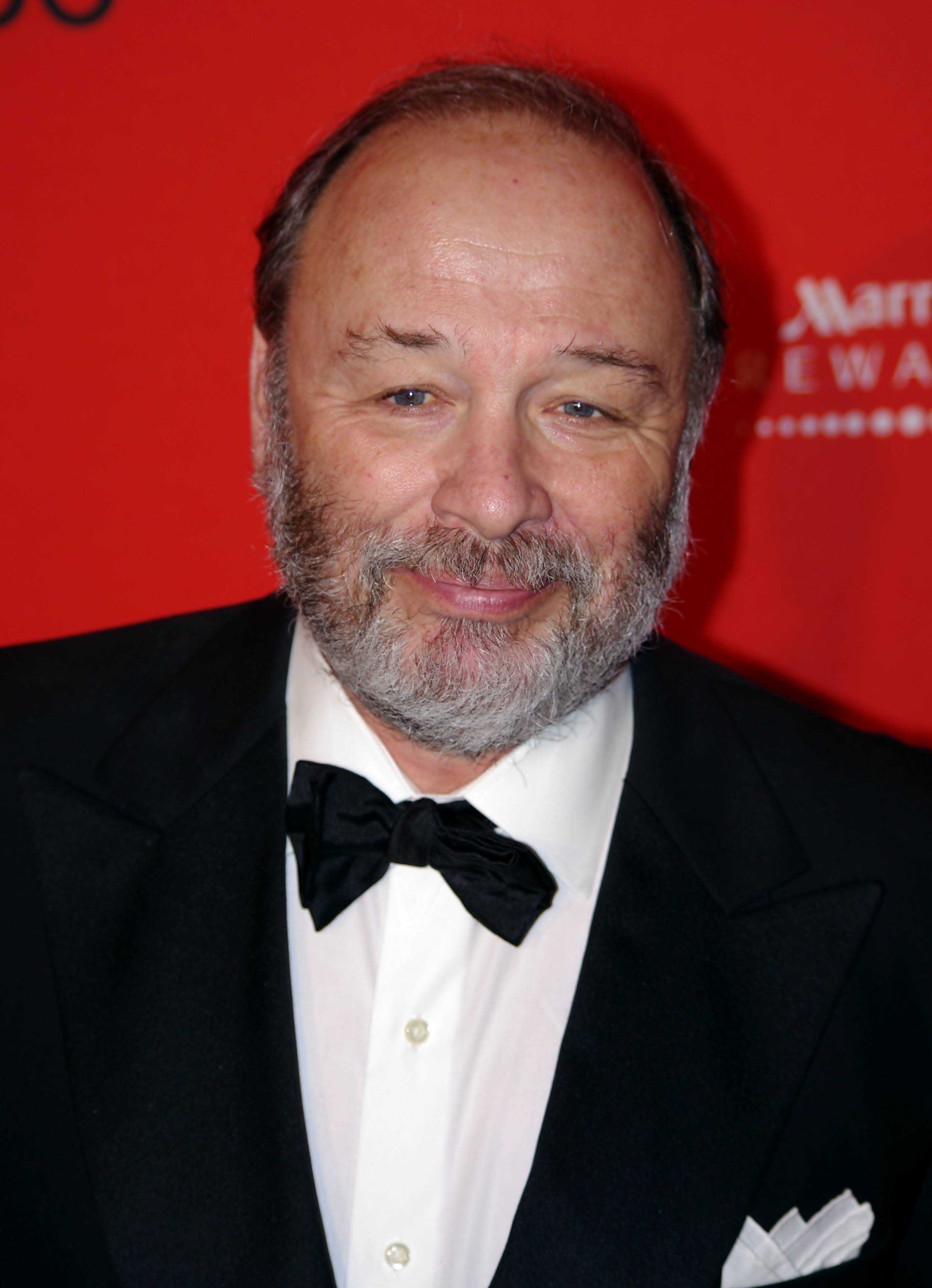This close-up photograph captures an older man, likely in his 60s, standing against a red wall with blurred white text displaying the letters "M-A-R-R." The man is dressed formally in a black tuxedo coat, buttoned up over a white button-up collared shirt with clear plastic buttons and a slightly crooked black bow tie. A crisp, folded white handkerchief adorns the front pocket of his jacket. He has a fair complexion, blue eyes, and exhibits signs of balding, with the front half of his head mostly bald and graying brown hair on the back and sides. A grayish-brown beard and mustache frame his face, which has a slight smirk and appears a bit shiny, likely due to the camera flash. The image gives the impression of being taken at a formal event, possibly resembling a red carpet occasion.